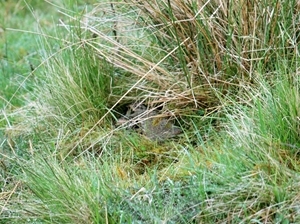A low-resolution, square, full-color photograph taken outdoors during the daytime, possibly for an animal or wildlife documentary. The image captures a natural setting with long, wild grass that varies from green to brown, with more brown concentrated in the center and upper right. Dominating the center of the photo is an animal burrow, which is darker than the surrounding grass. Inside this burrow, a small grey animal can be seen amongst the tall, straw-like grass blades, creating a sense of a hidden natural habitat.